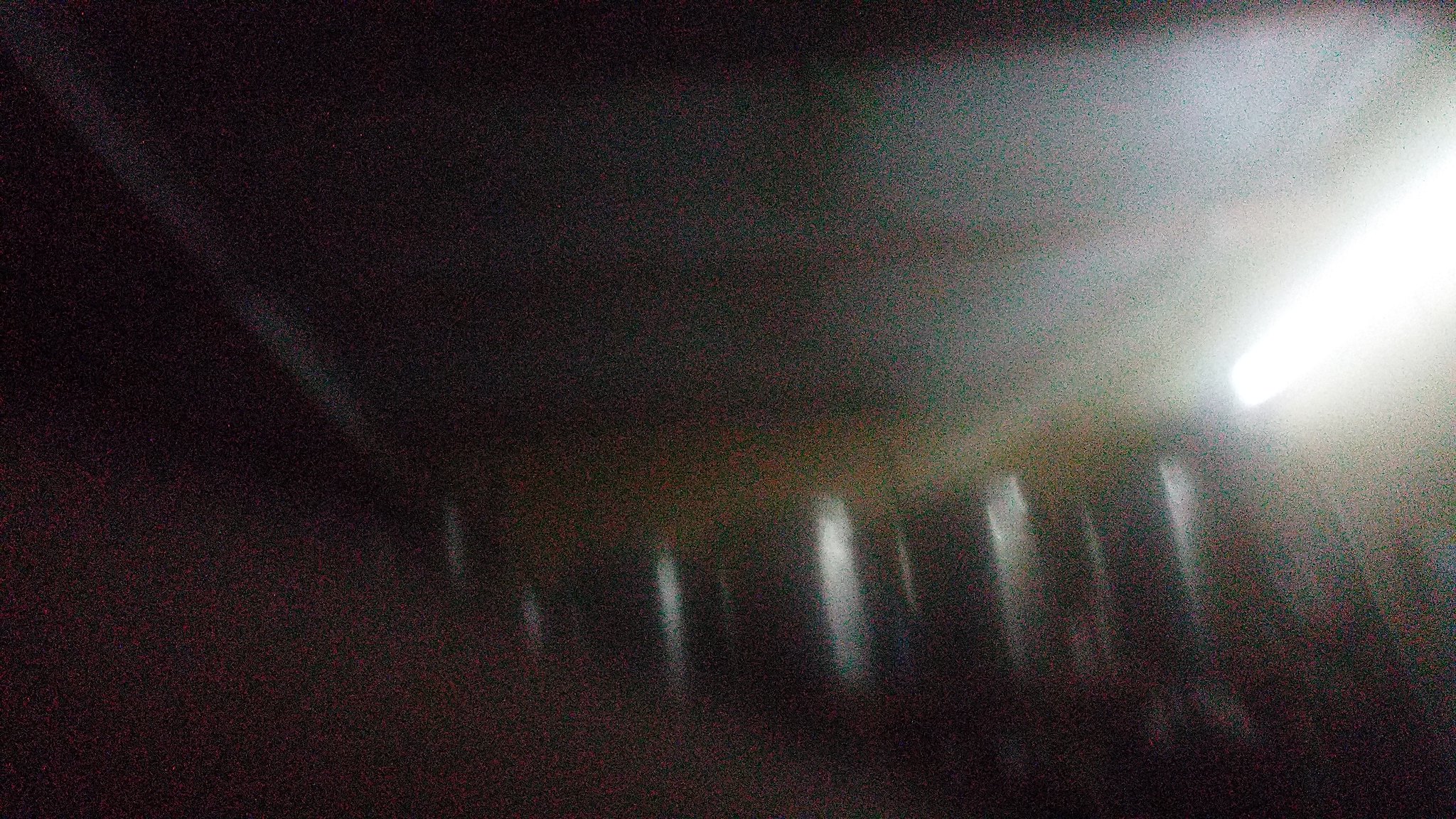This photograph appears to capture a dimly lit interior space, possibly a garage or carport. The scene is dominated by a bright, fluorescent white light in the upper right corner, creating significant contrast with the surrounding darkness and casting reflections on several metallic silver canisters. These canisters, which might be steel drums or large trash cans, are positioned on a shelf that runs along a yellow wall beneath a gray ceiling with visible beams. The image is heavily pixelated and grainy, with blurry elements, including a possible human finger in the lower left corner, contributing to an overall unclear and low-quality visual. The lighting imbalance and poor resolution make it difficult to discern additional details about the room or other objects within the photograph.